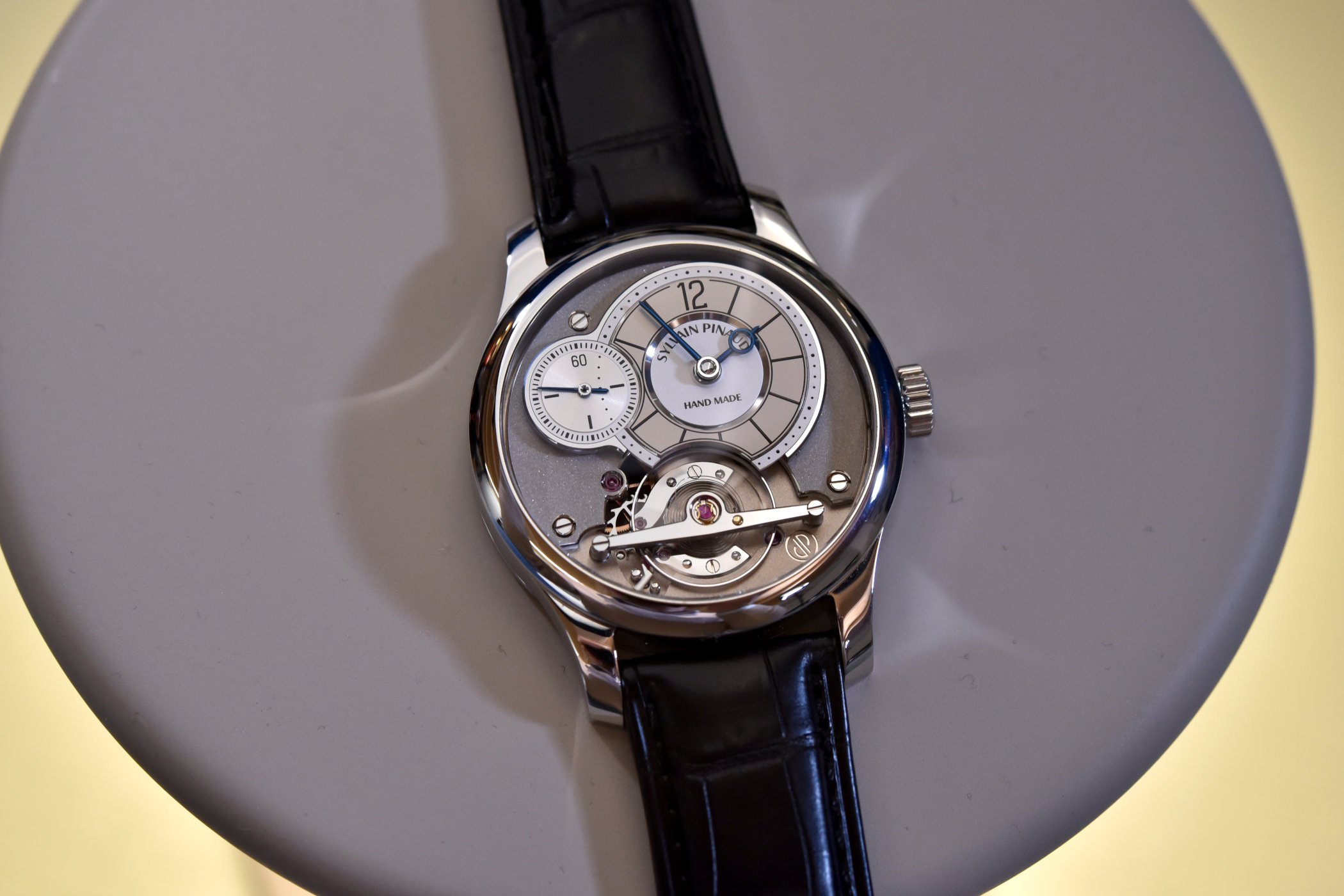The image depicts a wristwatch centrally positioned on a light gray, circular padded surface. The watch features a circular face with an analog clock on the right side, displaying the time at approximately 8:10, with blue hour and minute hands and the number 12 at the top. Inside the main circle, there are several additional circles, including a smaller one to the left that functions as a sub-dial with a 60 at the top, surrounded by numerous notches, likely for seconds. Below the main dial, intricate gears and a silver lever, part of the watch's mechanical movement, are visible. The watch is enclosed in a silver case with a knob on the right for adjustments, and it's attached to a black, possibly leather band, cropped out at the top and bottom edges. The watch face itself is cream to light brown in color, with the brand name in black, partially obscured by the watch hands, and the word "handmade" inscribed below. The overall composition is accented by hints of yellow on the outer edges of the photograph.